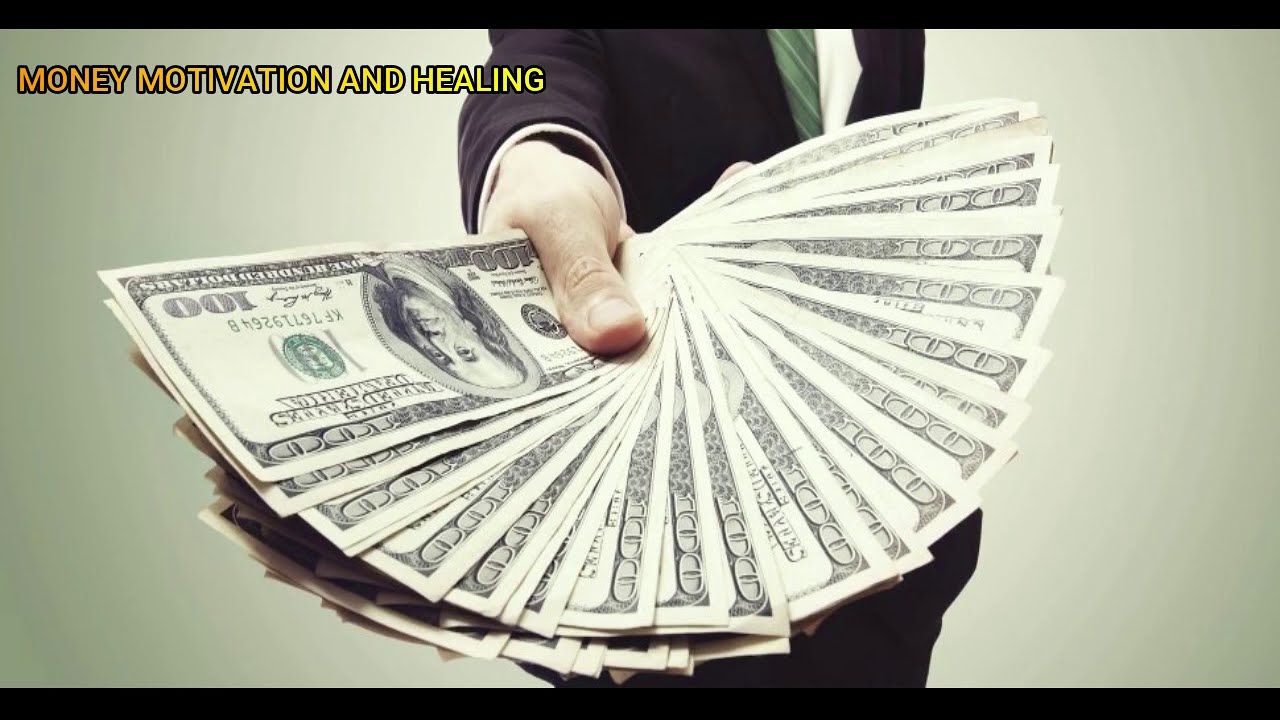In the image, a man dressed in a black suit, white shirt, and green striped tie stands against a grayish background. The top part of his body, including his head and shoulders, is not visible as the photo is cropped from his chest downwards. Prominently, he holds a fan of at least 20 fanned-out $100 bills, possibly totaling two to three thousand dollars, extending towards the camera. His thumb is visible gripping the money, clearly emphasizing the wealth he holds. In the top left corner, bold yellow text reads "money, motivation, and healing," adding a motivational context to the scene. The overall background subtly shifts in shades of gray.